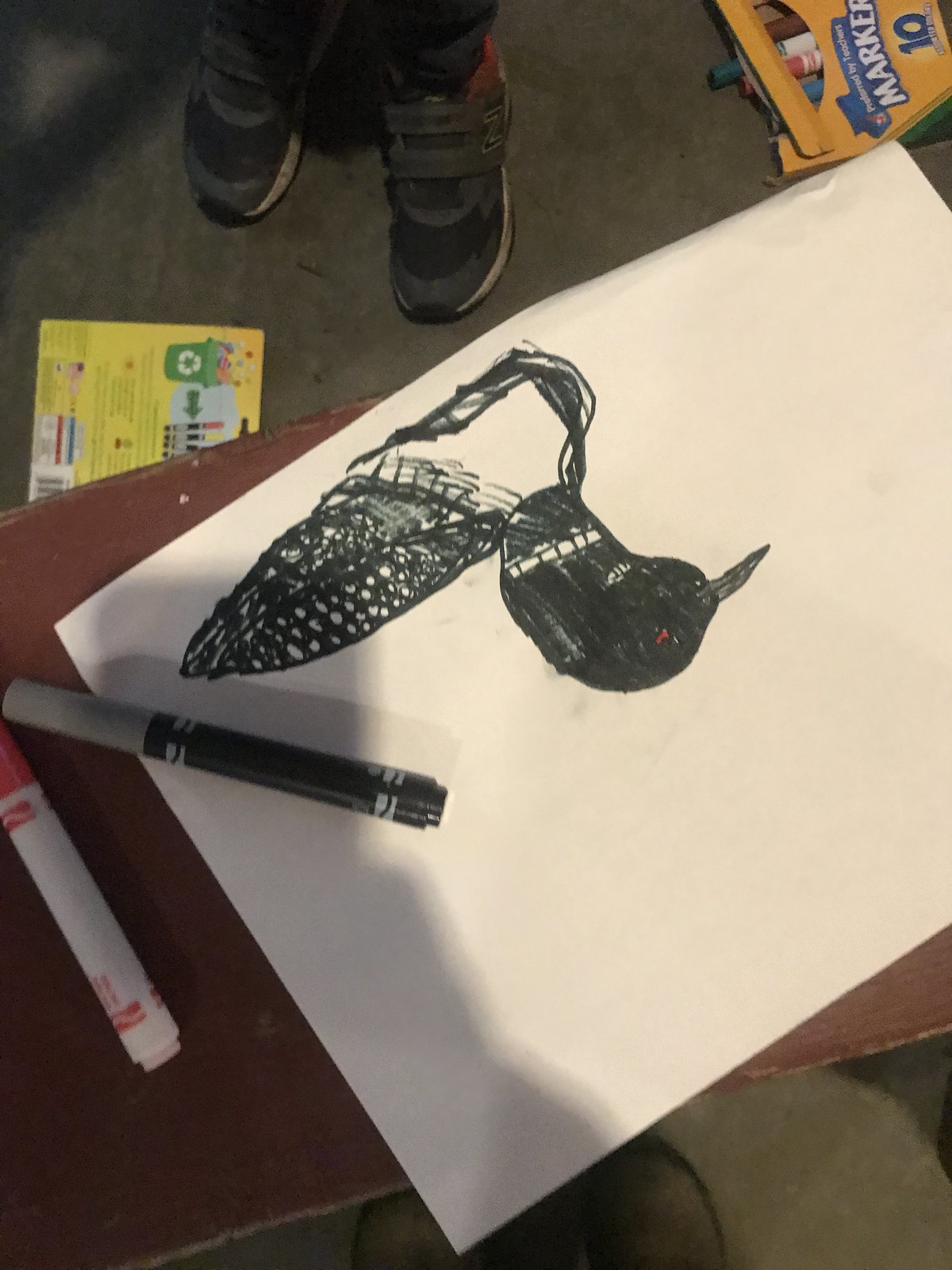In the center of the image lies a sheet of white paper featuring a hand-drawn duck rendered entirely in black ink, creating a monochromatic composition. The drawing rests on a small wooden table, flanked by two markers—one black and one red. Surrounding the table are various types of footwear. At the top are black sneakers with Velcro closures, while at the bottom sits a pair of tan boots. In the upper right corner, a box containing ten similar markers, including the black and red ones on the table, adds a splash of color and context to the scene.